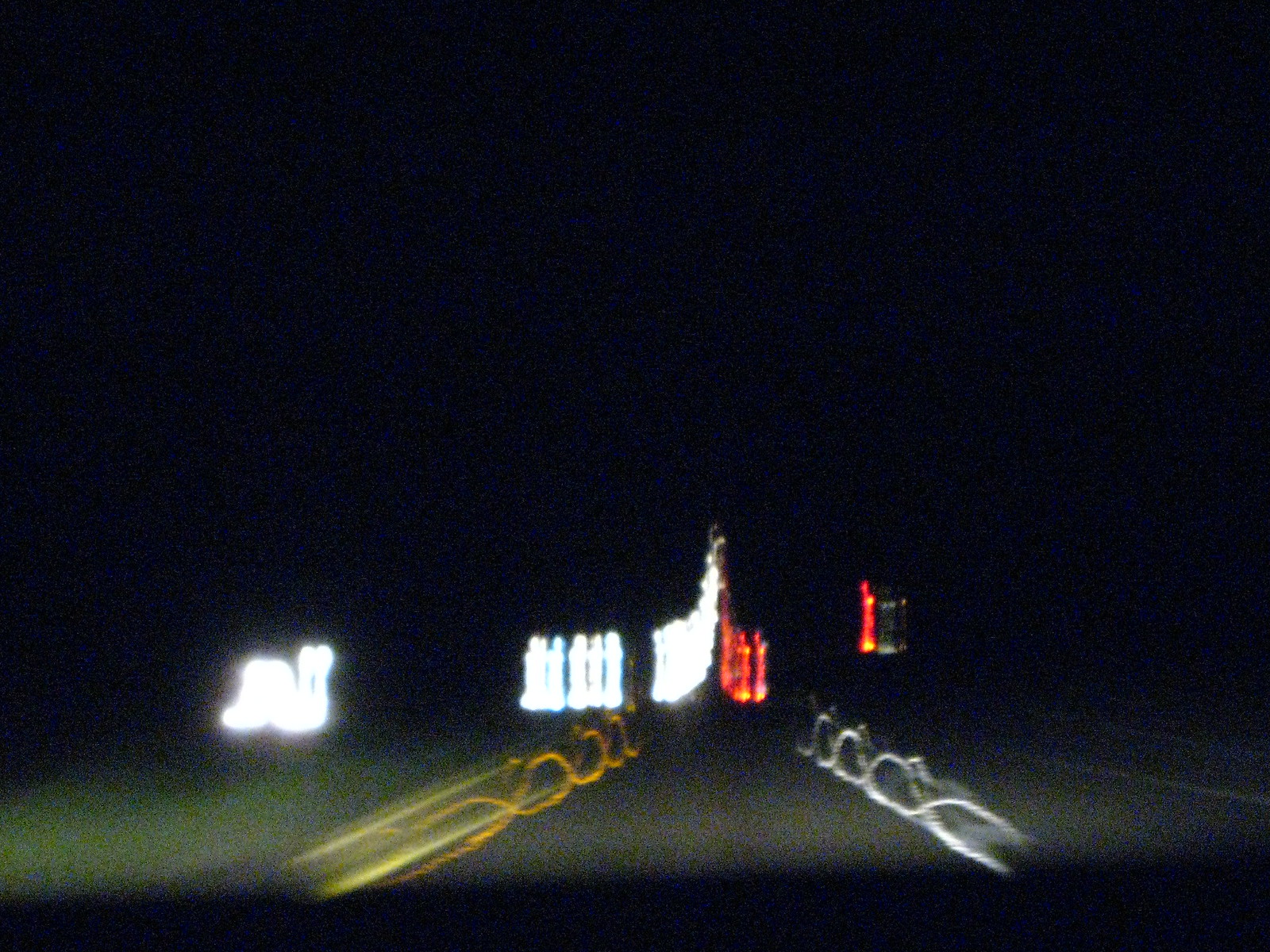This image, captured at night, shows a dark grey roadway accented by the blur of motion. The photograph's upper two-thirds is enveloped in darkness, while the lower third is illuminated by a dynamic display of lights and lines. On the left side of the road, a line of white lights stretches far into the distance, accompanied by a dark green grassy median. These white lights create an interlocking wave pattern as they trail off into the perspective. To the right, long red cylindrical brake lights mirror this wave-like formation, producing a visually striking effect. Yellow lines on the left and white lines on the right, both wavy due to the motion, add to the scene's sense of speed and direction. The photograph, taken from inside a moving car, captures the glowing trails of vehicle headlights and taillights, creating a mesmerizing, almost abstract visual representation of a bustling roadway at night.